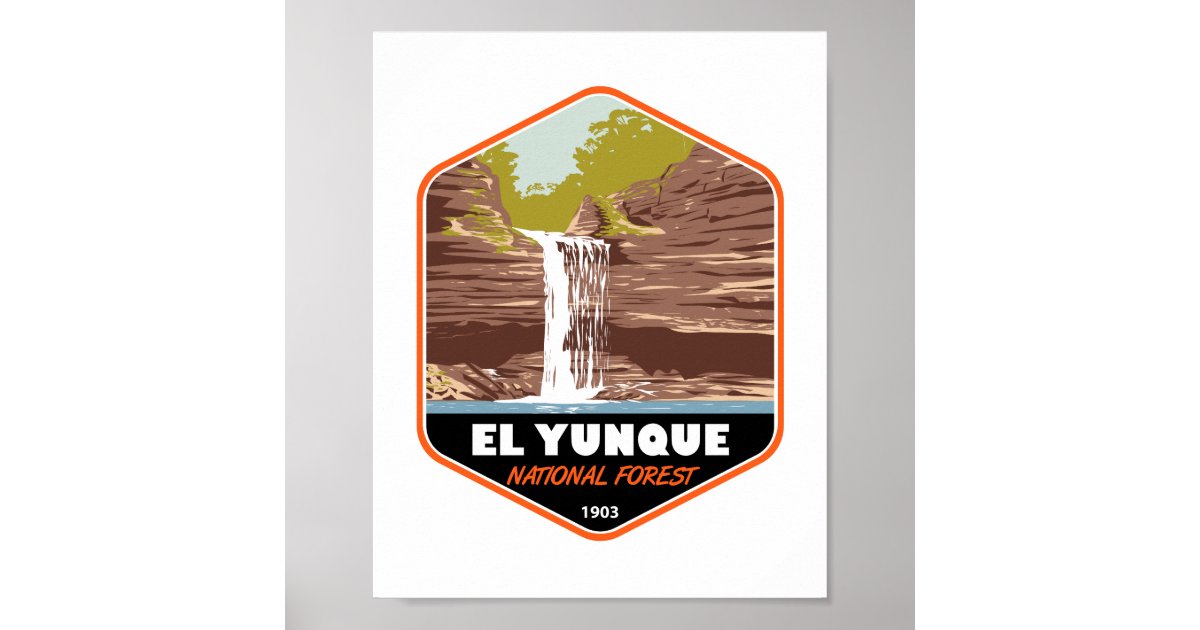The image is a square with a light gray border that is thinner at the top and bottom and thicker on the sides. Inside the border is a white background. Centered on the white background is a hexagon with rounded edges, outlined in orange, resembling a patch or a creative logo design. The top of this hexagon features a colored illustration of stony cliffs with horizontal strata layers, a waterfall cascading down the middle, and green trees at the top, indicating a natural landscape. Below the illustration is a bold blue line that spans from left to right. Beneath the line, in large white uppercase letters, is the text "LYUNQUE." Below this, in smaller orange letters, it reads "National Forest." At the very bottom of the hexagon, the year "1903" is written in white. The overall design uses simple, solid colors with no gradients, making it suitable for embroidery on a patch or similar application.